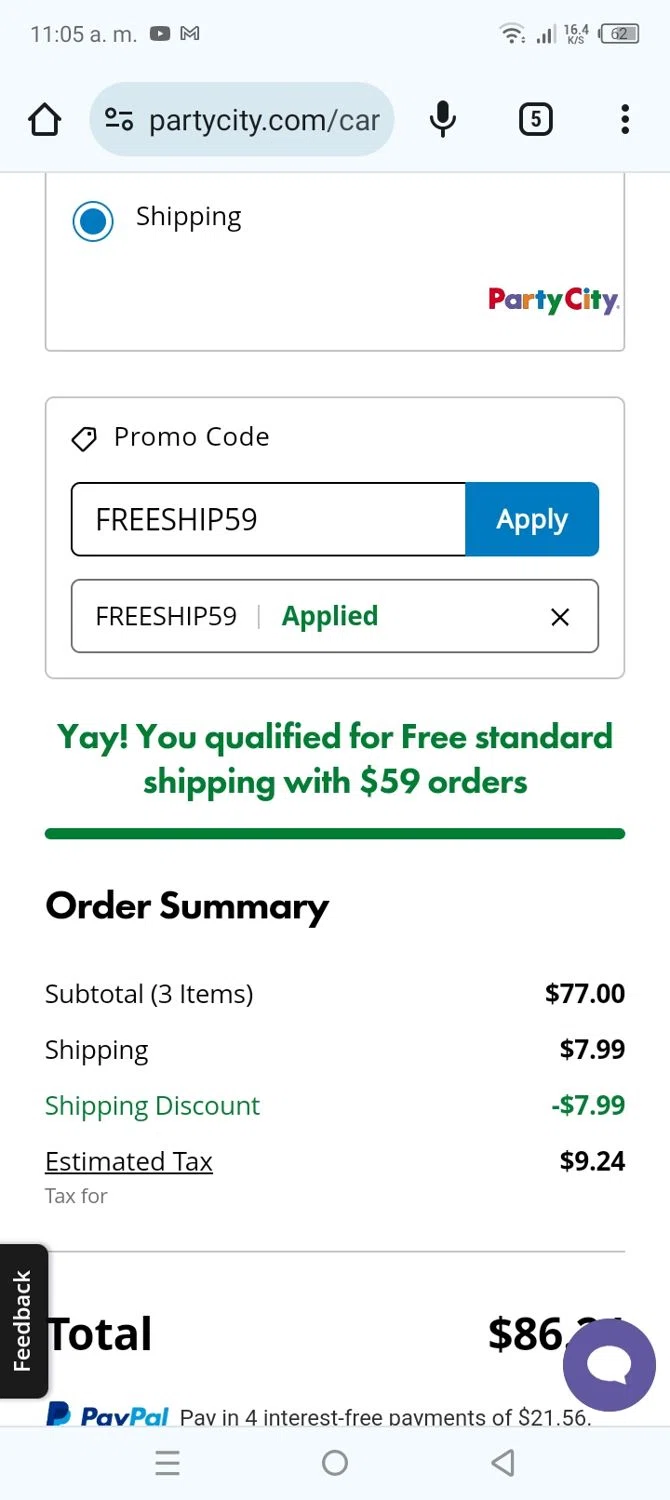A screenshot shows a smartphone screen captured at 11:05 a.m. with three out of four signal bars and about a quarter of the battery remaining. At the top of the screen, there's a home screen icon, followed by an address bar displaying "partycity.com/car". Next to the address bar is a microphone icon, a square with an 'S' in it, and a vertical ellipsis menu.

Below this section, there is a white rectangle with a gray border and the word "Shipping" beside a blue-highlighted, selected circle. To the right, the Party City logo is visible. Underneath, there is another white box with a gray outline containing the text "Promo Code" and a textbox filled with "Free Ship 59". A blue "Apply" button is next to it.

Beneath the promo code section, "Free Ship 59 Applied" is displayed in green text with an 'X' icon to the right. Below, it reads "Yay! You qualified for free standard shipping with $59 orders" in blue text. Finally, the screen shows an order summary stating "Subtotal (3 items): $77".